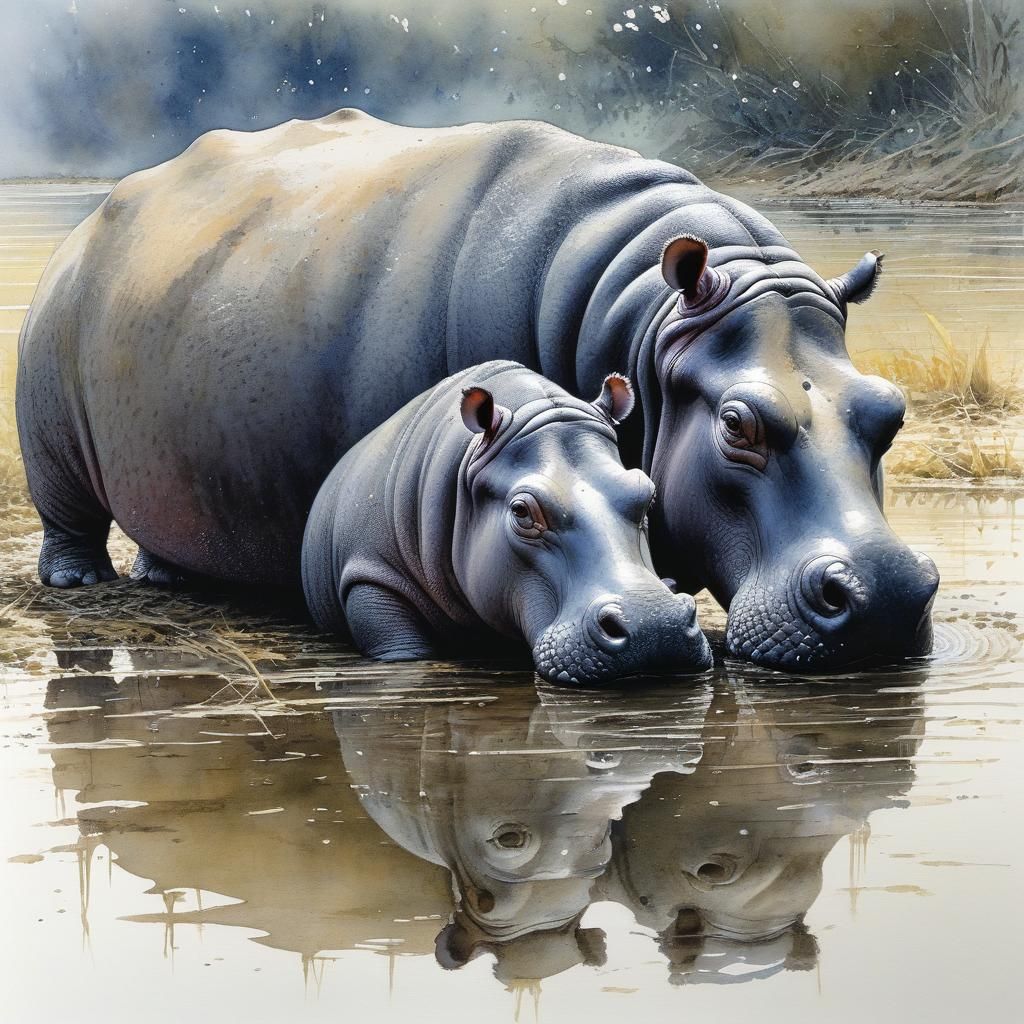The digital or AI-enhanced artwork depicts a serene scene featuring a mother hippo and her baby standing in murky water. Both hippos have their front legs and snouts submerged, while their reflective faces break through the surface, creating a mirrored image in the water. The mother hippo showcases a blend of gray and tan on her back hide, whereas both hippos overall bear steel gray coloring, with the reflected portions appearing much lighter. Their expressions are similar, with eyes directed slightly off-center towards the viewer. The background is a blurred mosaic of sparse grasses and scrub brush, lending a natural yet slightly stylized, almost dreamy quality to the setting. Flecks of white, potentially raindrops or bugs, add a touch of whimsy to the scene. The artwork is distinguishable by its unusual proportions and a slightly surrealistic touch, especially noticeable in the length of the hippos' legs and the overall color palette.